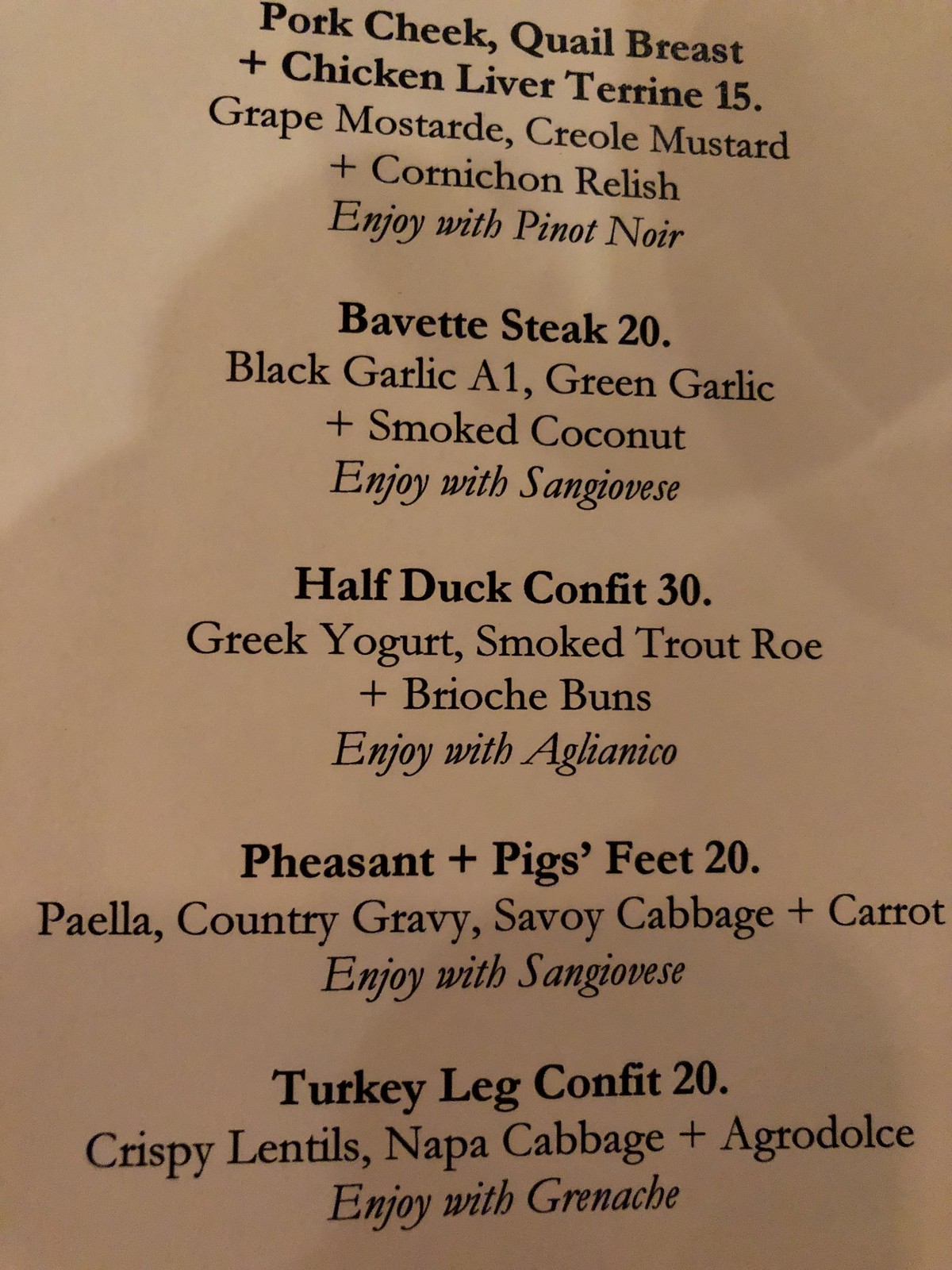The image displays a section of a menu page featuring gourmet entrees, written in black text on a light brown background. The menu lists five dishes, each accompanied by a price, key ingredients, and a suggested wine pairing. The first dish is a "Pork Cheek, Quail Breast, Chicken Liver Terrine" priced at $15, with ingredients like grape mustard, Creole mustard, and cornichon relish, recommended to be enjoyed with Pinot Noir. Next is the "Bavette Steak" for $20, which includes black garlic, A1 sauce, green garlic, and smoked coconut, paired with Sangiovese. The third item is "Half Duck Confit" at $30, served with Greek yogurt, smoked trout roe, and brioche buns, suggested with Aglianico wine. Following that is "Pheasant and Pig's Feet" for $20, featuring paella, country gravy, Savoy cabbage, and carrots, also paired with Sangiovese. The last dish is "Turkey Leg Confit" for $20, which includes crispy lentils, Napa cabbage, and agro dolce, recommended with Grenache.